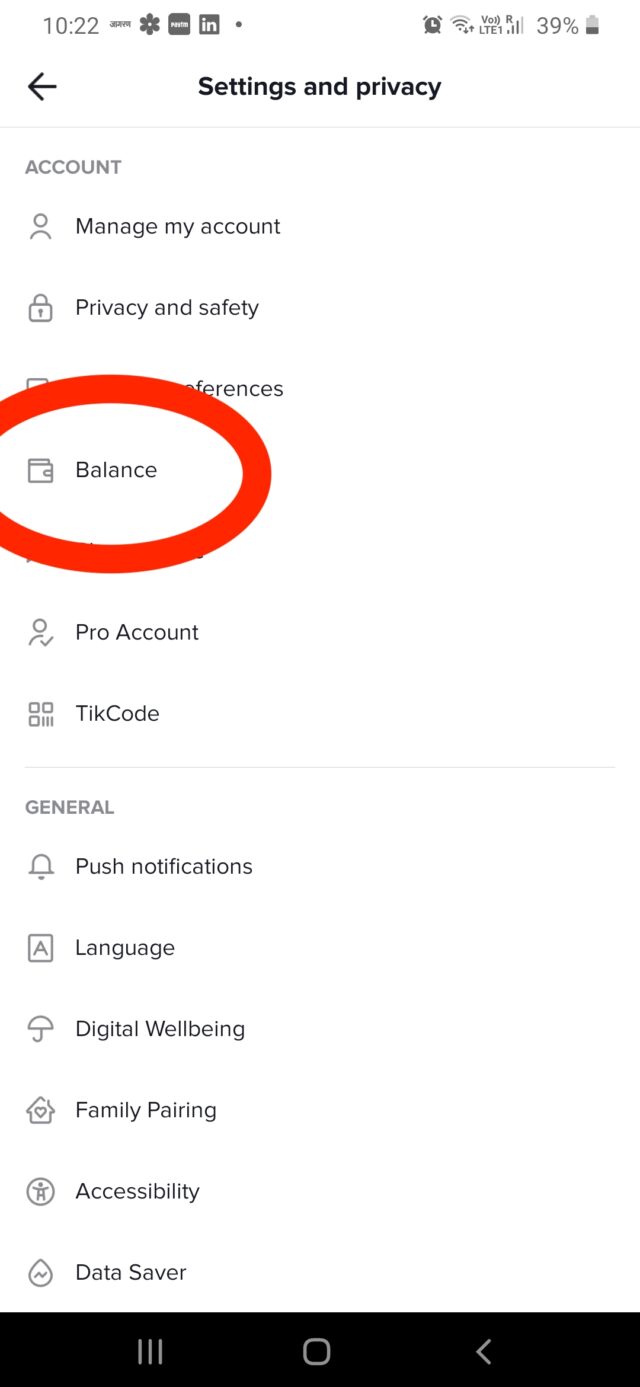Screenshot of LinkedIn Settings and Privacy Page

In this descriptive screenshot of a settings and privacy page, which appears to be from LinkedIn, the LinkedIn logo is prominently displayed at the top, accompanied by two other unreadable logos. The status bar includes a 39% battery meter, Wi-Fi icon, and an alarm clock icon. Below the status bar, a back arrow is located to the left of the text "Settings and Privacy."

The page is divided into two main sections: "Account" and "General." Within the "Account" section, the following options are visible:
1. A person icon labeled "Management Account."
2. A lock icon labeled "Privacy and Safety."
3. A partially obscured category with a red oval around it, showing an icon of a balance with a wallet.
4. Another category completely obscured by the same red oval.
5. A running person icon labeled "Pro Count."
6. Three squares and a bar icon labeled "Tick Code."

In the "General" section, the visible options are:
1. A bell icon indicating "Push Notifications."
2. An "A" within a square labeled "Language."
3. An umbrella icon labeled "Digital Well-being."
4. A house icon with a heart labeled "Family Pairing."
5. A child within a circle icon labeled "Accessibility."
6. An electric bolt within a drop of water icon labeled "Data Saver."

At the bottom of the page, there is a solid black bar containing a menu with three vertical bars, a square option, and a back arrow.